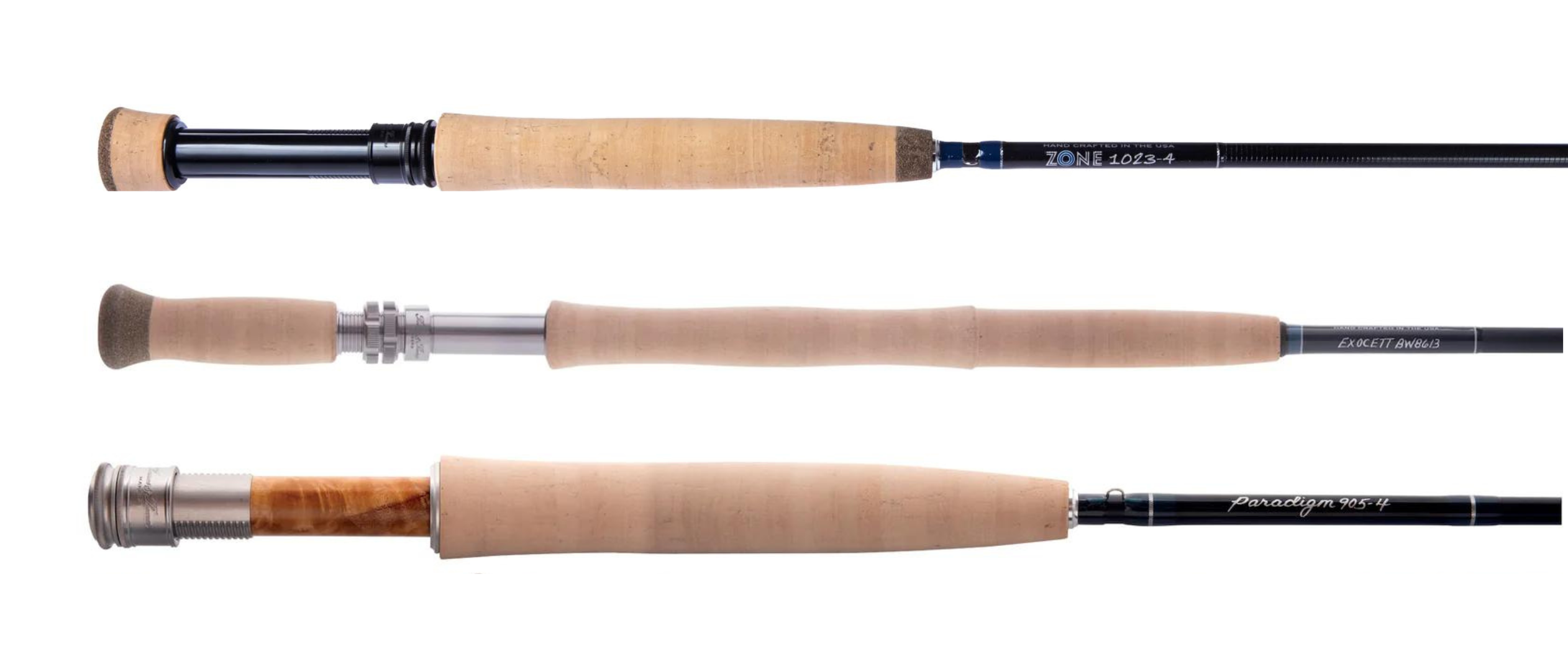The image showcases three horizontally aligned fishing rod sections, meticulously positioned one above the other against a stark white backdrop. The rods lack reels and text, emphasizing their structural details. The bottom rod features a silver base transitioning into a thick, wooden cushioned grip, followed by the pole. The middle rod consists of a wooden handle with a middle section of metal, then another grip area, and extends into the pole. The top rod presents a black handle with a wooden base, a cork area, and the rod which is black. The visible segments are likely from the upper parts of the rods, as only about a quarter length is displayed, leaving the hooks and full extent of the rods out of view. The overall focus lies on the varied materials and colors—including black, tan, light brown, dark brown, and silver—captured in this high-resolution, digitally placed presentation.